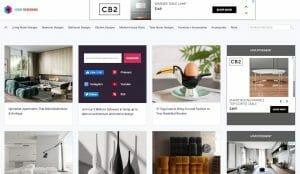This appears to be a screenshot of a shopping website or app displayed on a screen with a white background. The top section features an unreadable header label and a series of sub-menus beneath it, also too small to decipher. Below these menus, there are eight product images arranged in two rows of four. The small size of the images makes it difficult to identify the items clearly. The first image resembles a couch, while the second item might be a boiled egg holder. The third item appears to be a table, but the remaining images are indiscernible. This shopping platform seems to offer a variety of unrelated items, possibly indicating that it functions as a shopping aggregator for diverse products. The overall layout and design hint at a unique and eclectic selection of merchandise.